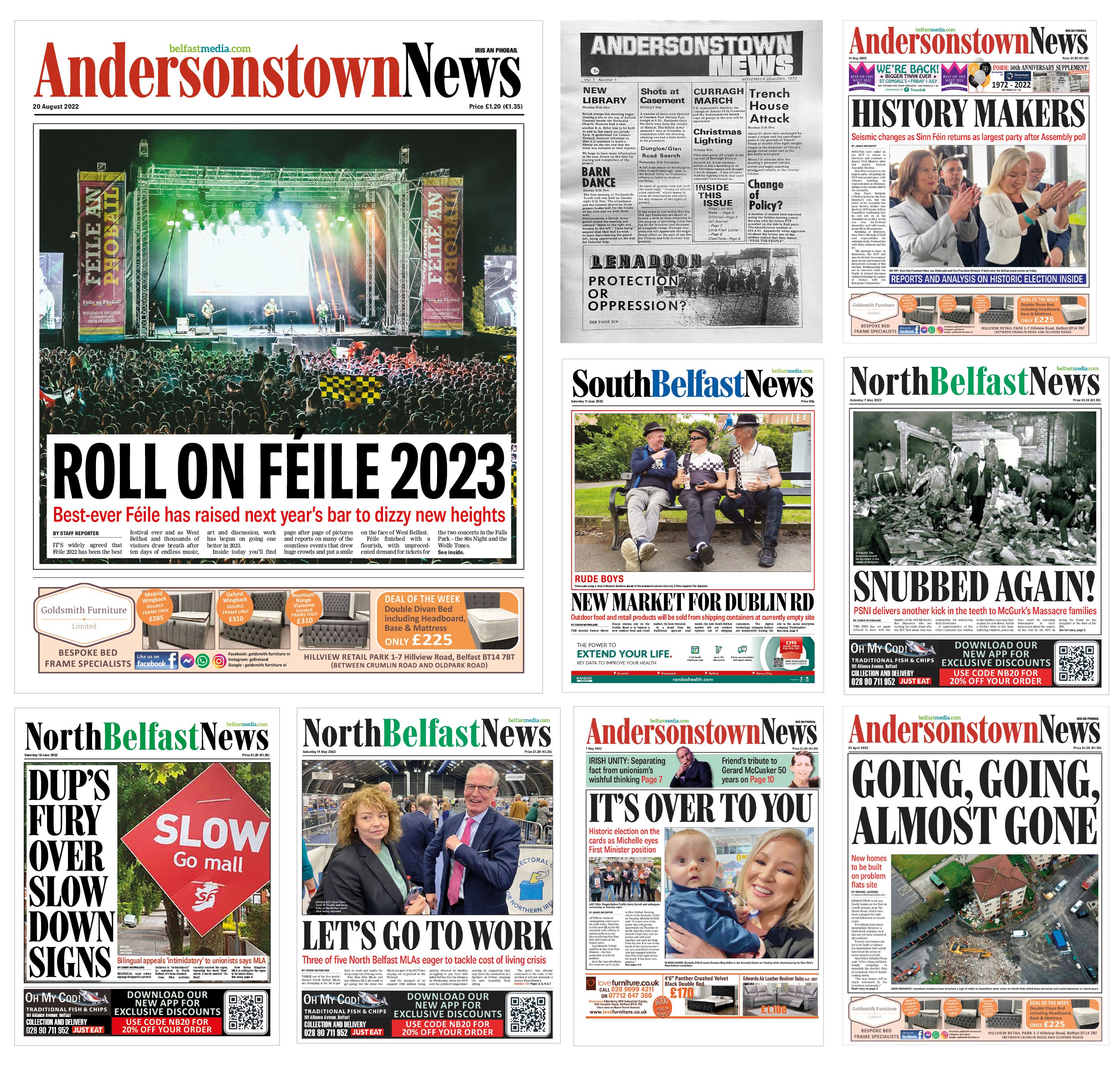The image showcases a variety of Northern Ireland-based newspaper front pages, arranged in a grid from top left to bottom right. Starting in the top left corner, the first front page is from the Andersonstown News, prominently featuring a headline about the Rollall and Field 2023 event. Adjacent to it is a black and white excerpt from an edition of the Andersonstown News, followed by a color version of the same newspaper to the right.

Moving to the second row, there is a noticeable shift in the newspapers. The first is the South Belfast News, and beside it, to the right, is the North Belfast News. 

In the bottom row, from left to right, there is another front page of the North Belfast News, followed by a consecutive cover from North Belfast News. Then, two front pages from the Andersonstown News complete the arrangement. 

The front pages cover a range of topics, predominantly political themes, with notable representation from Sinn Féin candidates. Michelle O'Neill is featured prominently on the front pages of two newspapers, and another Sinn Féin companion appears on the North Belfast News on the bottom row. Overall, the collection highlights the political landscape and issues relevant to Northern Ireland as reported by these regional newspapers.